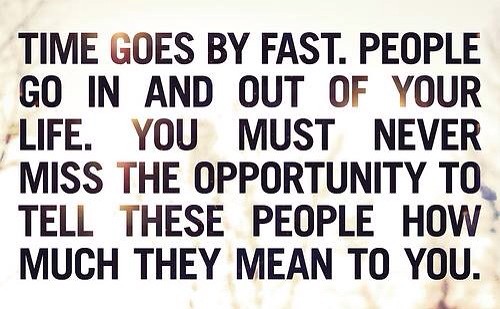The image features a detailed, inspirational quote designed in a landscape orientation. The background, predominantly beige with a marble effect and streaks of gray and rust, has a bright, sunny spot at the top, giving it a warm and luminous appearance. The background also includes a blurry, saturated overlay of yellow and blue hues that resemble sticks, which adds a layer of depth and texture. The central focus of the image is the bold, black sans serif text in all capital letters. The text spans five lines and reads: "Time goes by fast. People go in and out of your life. You must never miss the opportunity to tell these people how much they mean to you." This text occupies most of the visual space from left to right and top to bottom, making it the focal point of the design. The overall style blends illustration with graphic design typography, suitable for use as a background on devices, social media, or digital platforms, serving as a constant reminder of the importance of cherishing relationships.